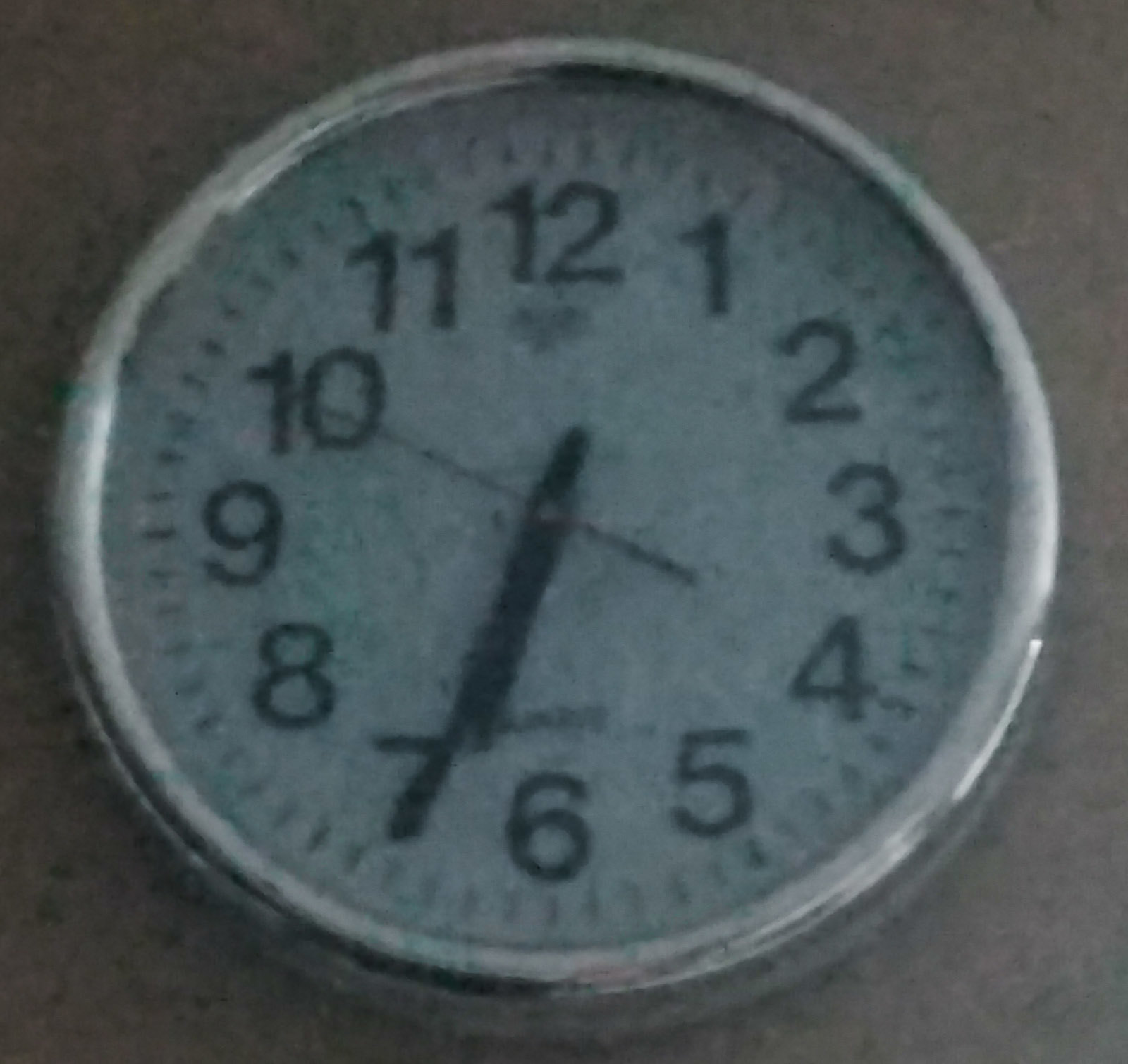This is a detailed, close-up color photograph of a round wall clock, displaying a slightly blurred and grainy texture. The clock is set against a greyish background surface that exhibits some black spots, which could either be imperfections or light artifacts. The clock features a silver metallic rim that catches the light at various points, specifically between the 9 and 10, 11 and 12, and 4 and 5 positions. 

The face of the clock is a greyish color with prominent black numerals ranging from 1 to 12. The hour and minute hands, both black, are positioned indicating a time of approximately 6:35. The hour hand is slightly to the right of the 7 marking, while the minute hand points directly at 7. Additionally, there is a slender black second hand centered at the 10-second mark. 

A blurry logo is faintly visible under the numeral 12 and above the numeral 6, adding to the clock's design details. Overall, the reflections and minor details, despite the blurriness, contribute to the rich character of the image.